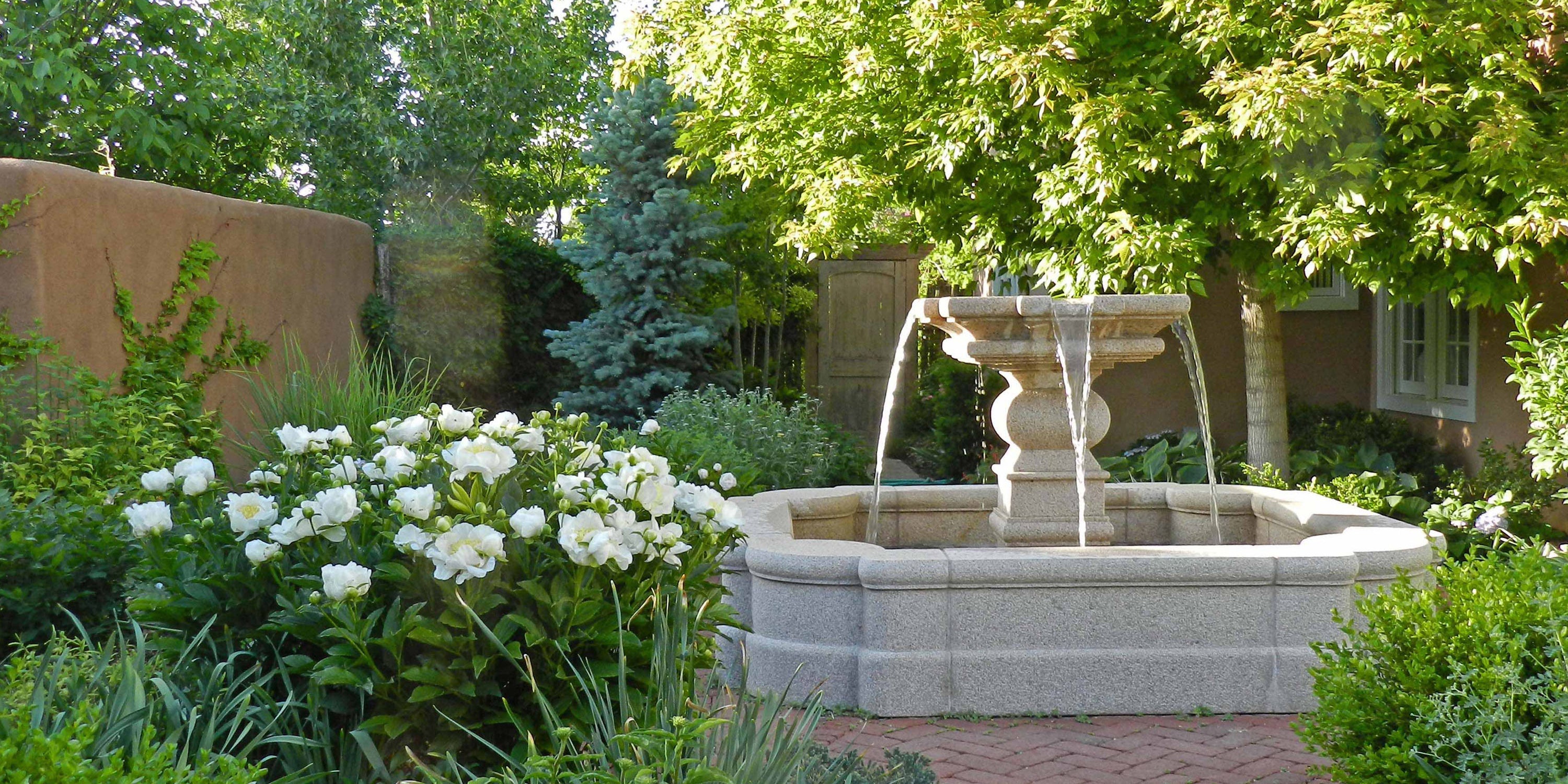The image captures a serene backyard in a landscape layout, dominated by lush greenery that envelops the scene. In the foreground, there's a chevron-patterned red brick walkway leading to a central concrete fountain. The fountain, square-shaped with decorative curved edges, features a cylindrical column that fans out at the top and has four streams of water pouring from its elevated platform. 

On the left side of the image, a large, rust-colored wall—almost reddish-tan—stands behind a mix of trees, bushes, and a cluster of white flowers. The right side reveals a sizable, partially obscured house with a tannish façade and white windows, set underneath a canopy of trees, including one notably large tree near the house's corner. 

Surrounding the fountain are diverse plants, bushes, and a collection of evergreen trees on the far left. The scene, bathed in the soft light of either morning or evening, evokes the charm of a secret garden, with a sense of tranquil seclusion punctuated by the gentle sounds of flowing water.